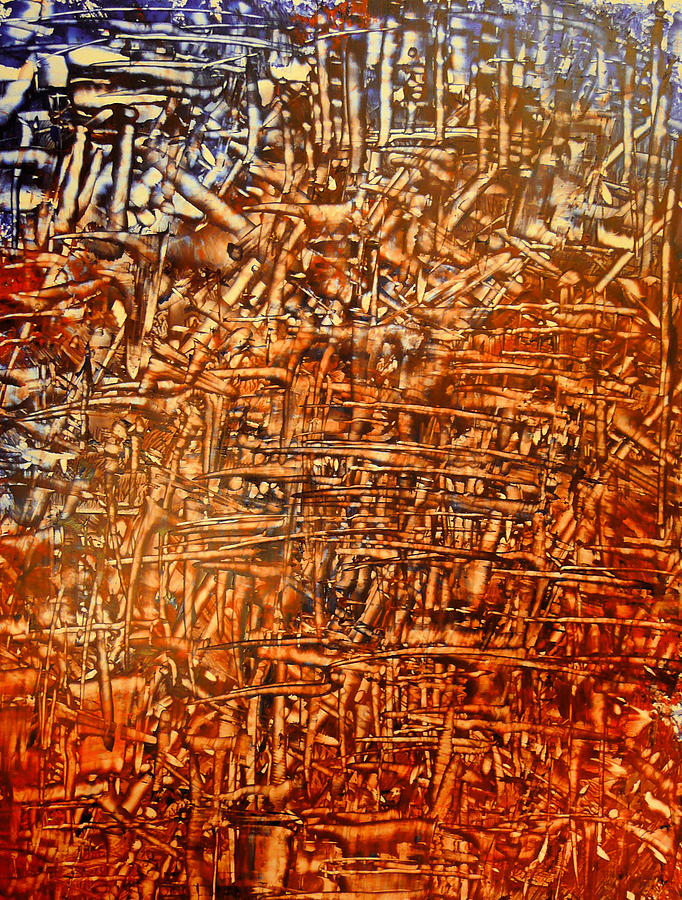This image is a close-up of an abstract painting, predominantly featuring a reddish-orange, rusty color palette. The painting is dense with intricate patterns and shapes that resemble various industrial elements, such as curved pipes, cylindrical components, and zigzagging lines. In the upper left corner, you can spot a mix of black and white hues, while the upper right corner showcases hints of purple and yellow. Additionally, there are blue hues scattered towards the top, providing a stark contrast to the warmer tones. Upon closer inspection, there appears to be a shape resembling a finger in the bottom left, adding an element of intrigue. The background behind these abstract shapes is white, making the vivid and complex details stand out even more distinctly. The overall effect of the painting is both wild and concentrated, invoking a sense of chaotic beauty.